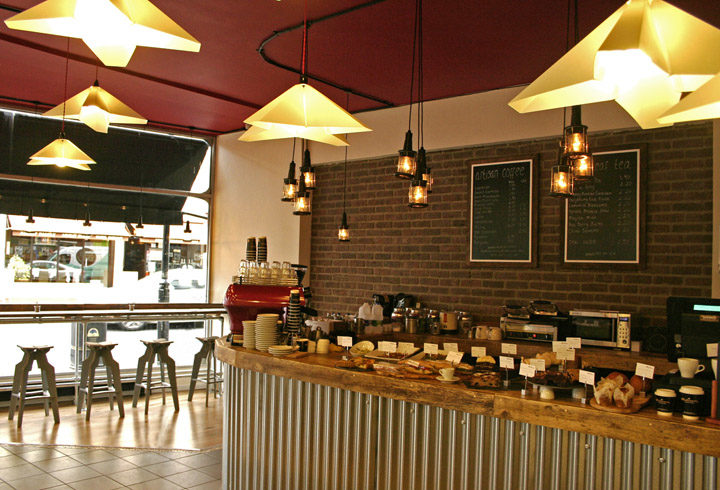The photograph captures the cozy interior of a small coffee shop bathed in a mix of natural and artificial light during the daytime. Dominating the upper portion of the image, the ceiling is painted red and adorned with distinctive star-shaped, white-tannish chandeliers. Below, a counter spans the scene, featuring a wooden countertop and a corrugated metal front. An array of enticing pastries, each labeled with a small note card, are displayed prominently on the counter, alongside various coffee machines, a toaster oven, and a microwave.

To the left, a large picture window offers a view of the street outside, accompanied by a long table and four stools positioned beneath. The right side of the scene is marked by a striking red brick wall, which serves as a backdrop for two framed blackboards displaying the menu, though the writing is too distant to discern. The ambient charm created by the interplay of light, eclectic decorations, and the rich textures of wood and brick evokes a warm, inviting atmosphere typical of a beloved local cafe.